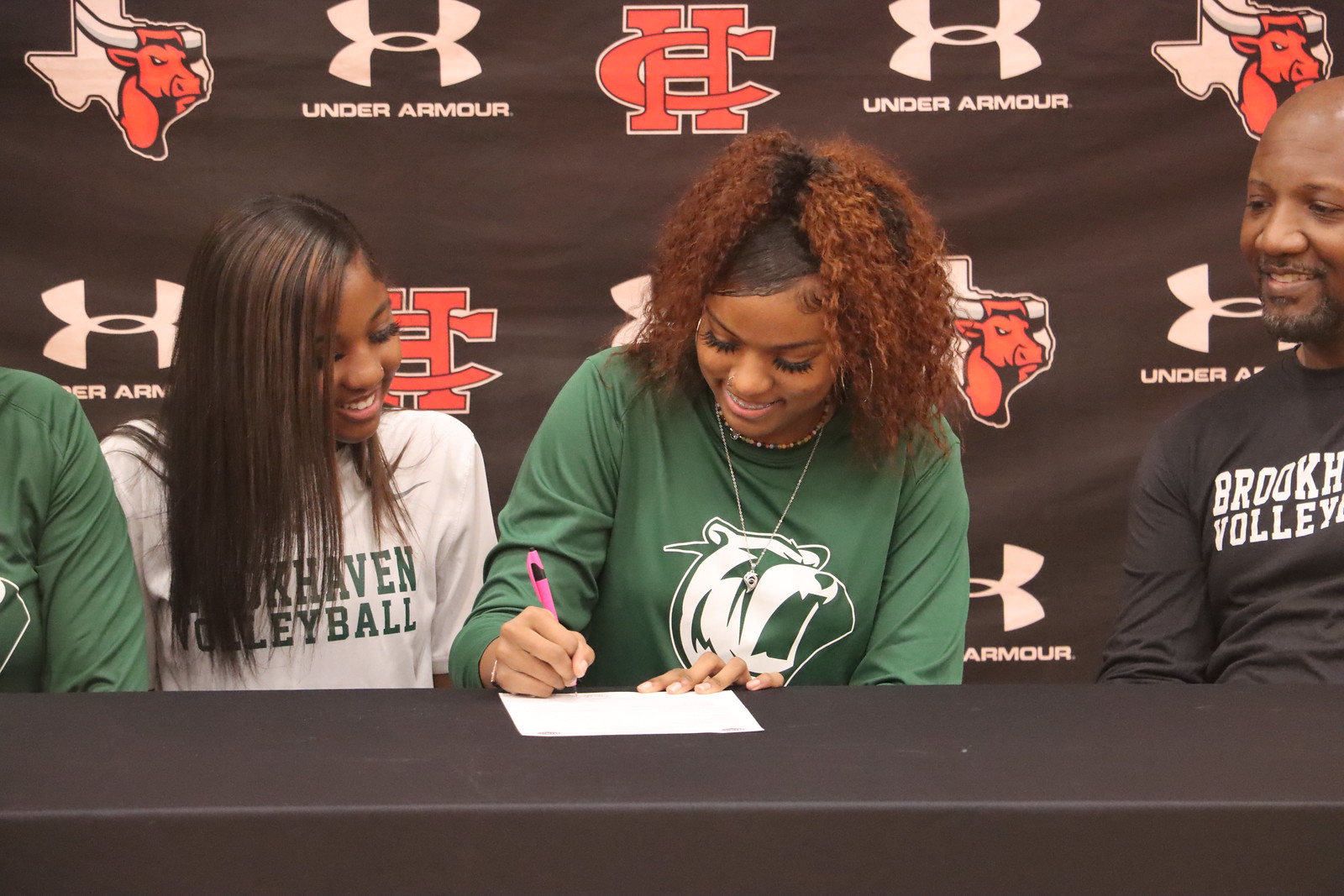In the photograph, a pivotal moment is captured at a black table where a young woman is signing a document. She is wearing a long-sleeved green shirt adorned with a white logo of a roaring bear. The signing is being done with a pink pen held in her right hand. Her reddish-black hair cascades down as she focuses intently on the task. To her left, a young woman with long black hair, dressed in a gray short-sleeved shirt that reads "Brookhaven Volleyball" in green text, watches and smiles. On the far right, a man in a long-sleeved black shirt with "Brookhaven Volleyball" written in white text is looking down at the document being signed. Positioned behind them is a black backdrop displaying various logos, including a red bull inside a Texas outline, a Thunder Armor logo, and another logo with the letters "CH." An arm appears on the left side of the photograph, partially cut off by the edge. The ambient feeling suggests a proud and significant event, possibly the young woman's commitment to joining a school team, surrounded by support and joy.